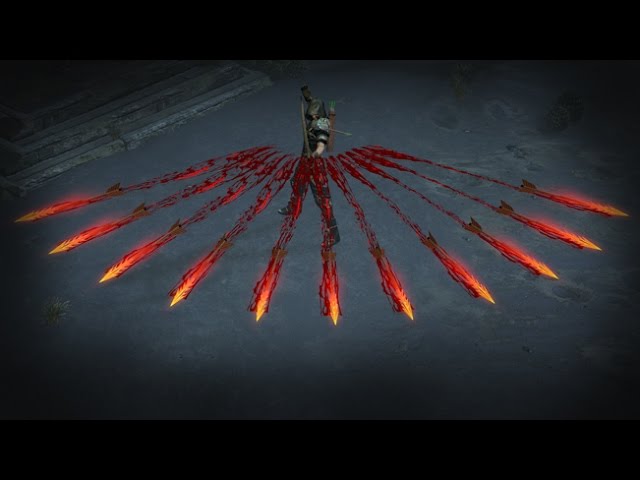In this digital image, which appears reminiscent of a video game screenshot, a hooded archer stands against a very dark gray background, almost resembling the surface of a mysterious planet. The archer, with pale white or olive-toned skin, is adorned in a green hood and armor, and wears dark boots. A brown quiver rests on their back, filled with arrows that feature green fletching. They hold a bow in their hand, partially visible as a vertical line next to their head. The focus of the scene is a special ability being activated: eleven arrows are fanning out in a dynamic, fiery display from left to right. These arrows start as dark red near the archer and progressively lighten, glowing like flames toward the viewer. The upper and lower edges of the image are bordered in black, enhancing the dramatic effect of the archer’s powerful maneuver. A gray stone platform can be seen below the archer, with a raised gray stone structure in the upper left background, adding depth and context to the setting.